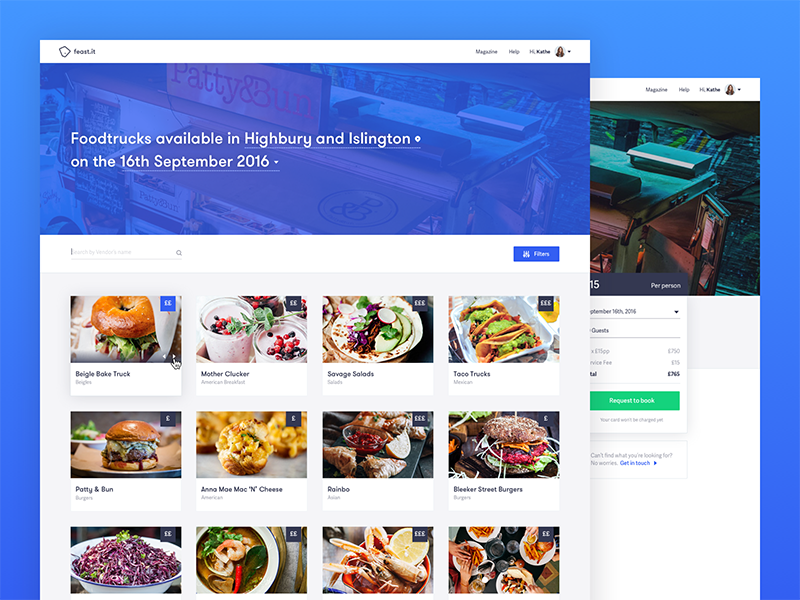Set against a blue background, this image features two prominent pop-up boxes displaying screenshots. The clearly visible upper box has a white banner, while the lower one features a blue banner depicting what appears to be a restaurant counter with the text "Patty and Bun." Below this, white text announces, "Food trucks available in Highbury and Islington on the 16th September 2016." 

In the upper right corner, there is a blue action button labeled "Filters." Beneath the banners are three rows of food images against a white background, showcasing various food truck options. 

For instance, in the upper left corner, there's an image of a bagel sandwich labeled "Bagel Bake Truck." To its right, an image of two berry smoothies is accompanied by the text "Mother Clucker." Further to the right, a plate of salad is shown, labeled "Savannah or Savage Salad." Finally, in the upper right corner, there's an image of a tray of tacos topped with beef and shredded lettuce, marked "Taco Trucks."